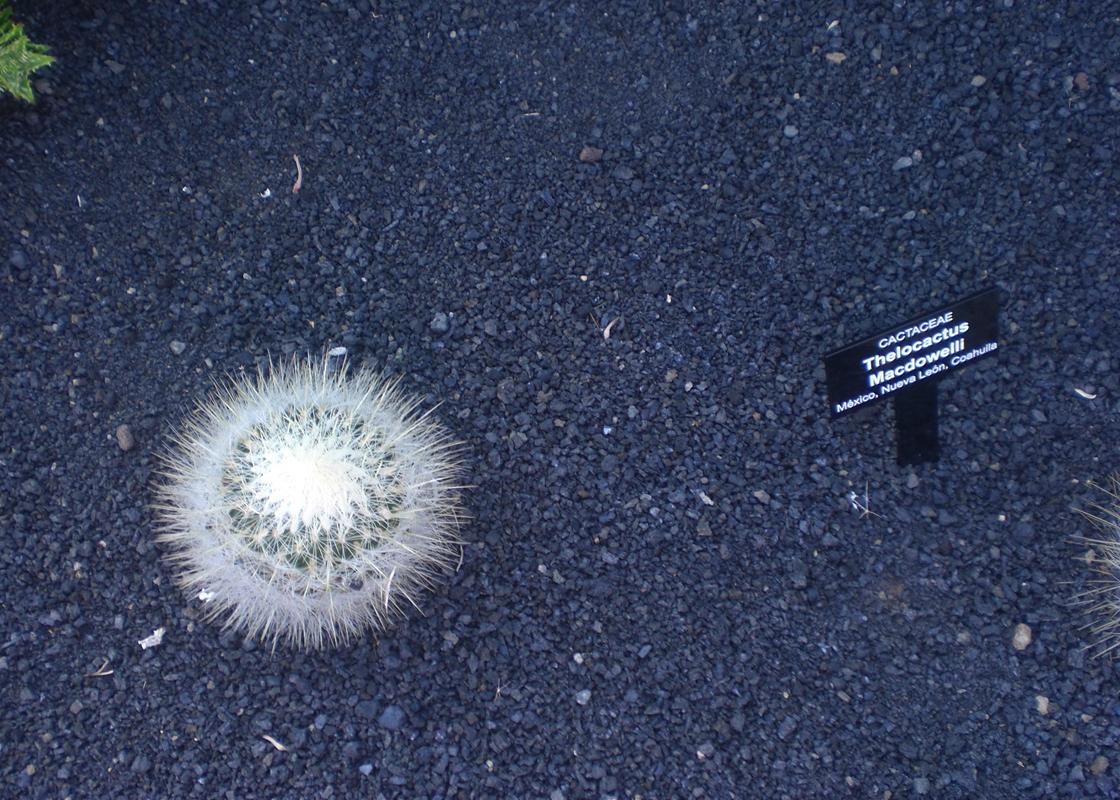The image depicts an outdoor garden scene in the middle of the day, characterized by a ground surface covered in dark gray, stone pebbles resembling an unfinished roadway. Dominating the lower left corner is a distinctive round cactus, notable for its long, yellowish, furry spines and a top section that appears almost completely white. The cactus is green at its core but gives off a whitish appearance due to the dense spines. In the upper left corner, a small green plant is partially visible, while another partly cut-off cactus is seen to the right. A small rectangular black sign to the right of the central cactus reads, "Cactaceae, Ferocactus Macdowell, Mexico, Nuevo León, Coahuila," providing identification and origin details. The setting appears to be outdoors, likely in a curated garden space.